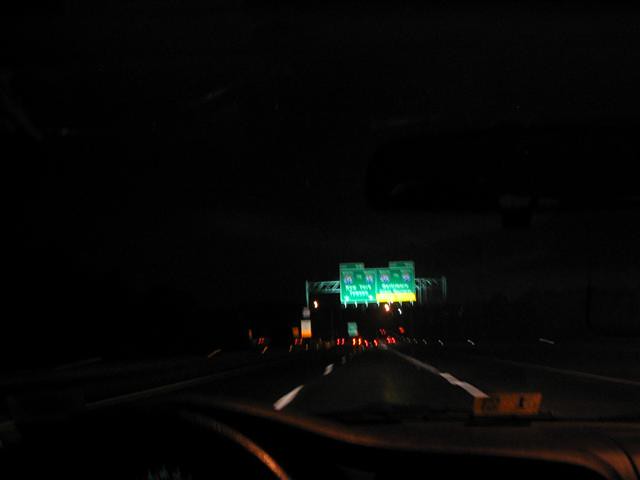Captured from inside a moving car at nighttime, this image portrays a dimly lit highway scene under a pitch-black sky. The view through the windshield is notably blurred, with faint traces of an orange sticker visible on the glass. The roadway features multiple lanes, and ahead, the glowing red taillights of at least four cars can be seen, indicating moderate traffic. Overhead, a collection of green highway signs with white text provide directional information. Despite the blurriness, the classic yellow and blue symbols and exit numbers are partially discernible, suggesting navigation options. The signage appears to indicate different destinations depending on whether one takes the exit lane or continues straight, though the specific text is illegible due to the image quality.